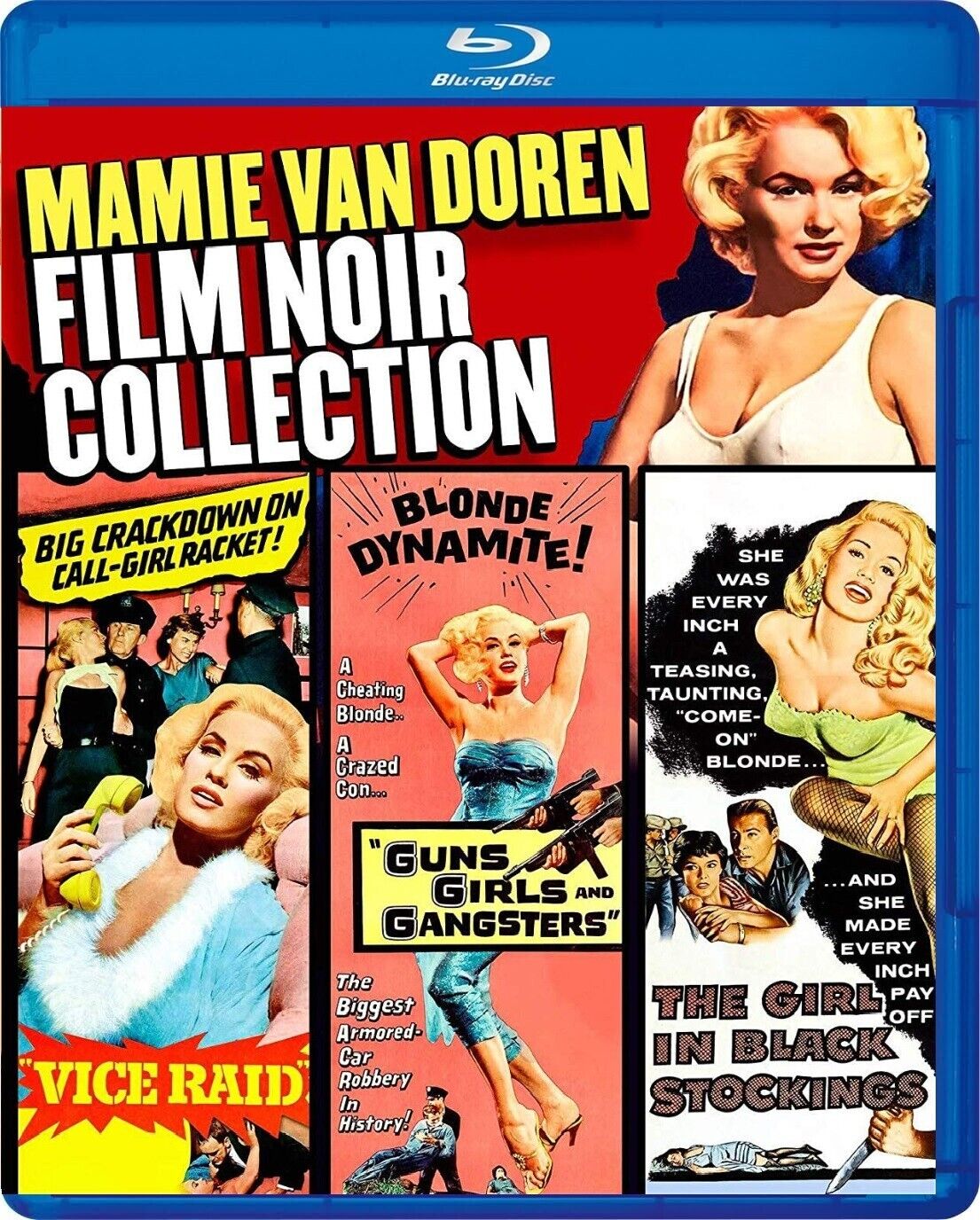The Blu-ray Disc cover showcases the Mamie Van Doren Film Noir Collection. Dominating the cover, the title "Mamie Van Doren" is rendered in bold yellow text, followed by "Film Noir Collection" in white underneath. On the right side, a prominent image of Mamie Van Doren, a classic blonde beauty, enhances the vintage aesthetic. Below this, the cover features three vertical rectangular panels, each representing a different film.

The first panel, titled "Vice Raid," depicts Van Doren with a 60s hairstyle, wearing a blue robe with a feathery outline, emphasizing a headline: "Big Crackdown on Caldwell Racket." Police officers and women in the background hint at a tumultuous scene.

The central panel, "Guns, Girls, and Gangsters," bears the proclamation "Blonde Dynamite" and describes "the biggest armed car robbery in history." Here, Van Doren strikes a dynamic pose in a blue jumpsuit and heels, her arms lifted and eyes engaged with the viewer, surrounded by illustrations of machine guns.

The final panel, "The Girl in Black Stockings," portrays Van Doren in a provocative green outfit and black stockings, her hair longer, against a backdrop of a sinister scene with a nervous couple, a hand clutching a knife, and a body lying presumably lifeless.

This detailed, stylistic cover art encapsulates the allure and drama of Mamie Van Doren's classic film repertoire.